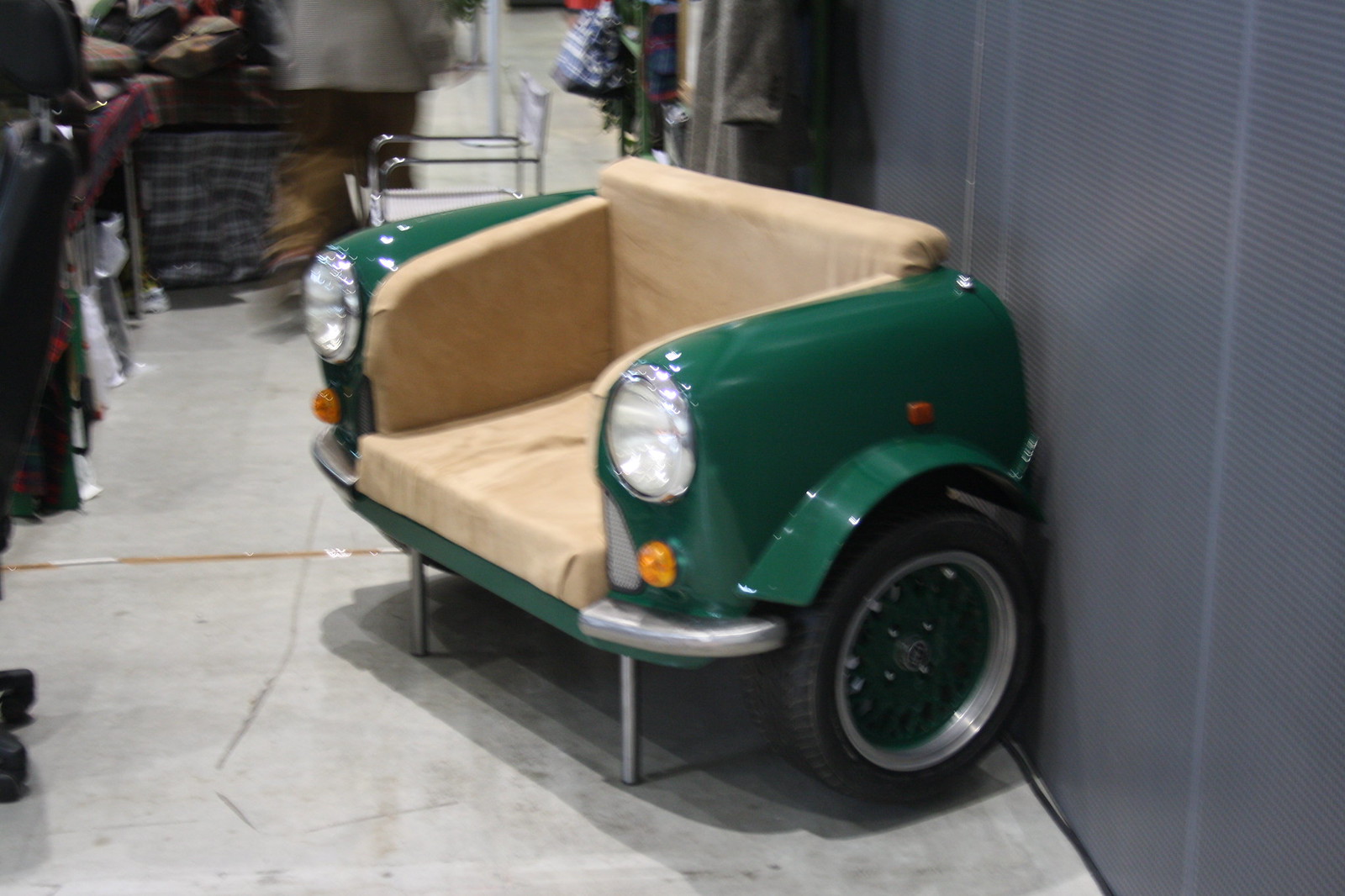This photograph captures a somewhat blurry backstage area or garage-like setting, cluttered with various items including a desk, chair, and other bric-a-brac. Prominently centered is a novelty loveseat fashioned from the front end of a Mini Cooper, British in origin. The car front, painted dark green, features round headlights that have been ingeniously repurposed into armrests. The tan seating area is nestled in the middle, between the headlights. The cut-off section behind the front wheels seamlessly transforms into the backrest of the sofa. The ground is a stone concrete path, and several random objects are scattered around, including a person walking with a cart. The overall impression is a creative piece likely used as a prop for theater performances or similar environments.